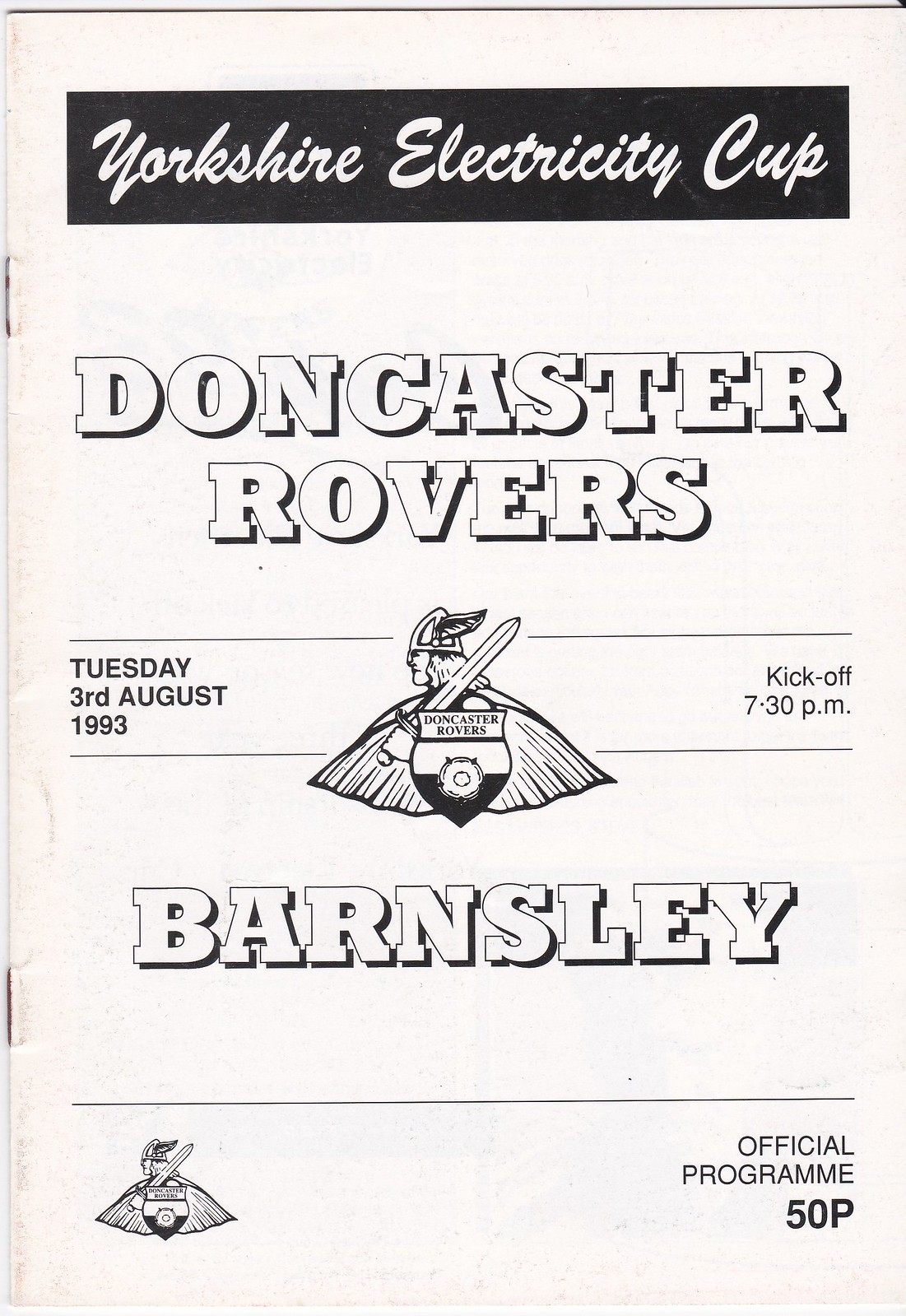The image is a scanned, printed page from a booklet or advertisement, primarily white with black ink designs and text. At the top, there's a large black rectangle with "Yorkshire Electricity Cup" written inside in white cursive. Below this, "Doncaster Rovers" is displayed in large block capital letters. Central to the design, there is a logo featuring a Viking with a winged helmet, holding a broadsword over his shoulder, and a cape billowing out dramatically. Superimposed on the Viking is a crest with the words "Doncaster Rovers" in black and white. To the left of the Viking logo, it states "Tuesday 3rd August 1993," and to the right, "Kickoff 7.30 p.m." Beneath this, "Barnsley" is prominently displayed in capital letters. Towards the bottom left of the page, a smaller version of the Viking logo is situated. On the bottom right, it reads, "Official Program 50p." The page is held together by two slightly rusty staples on the left side.